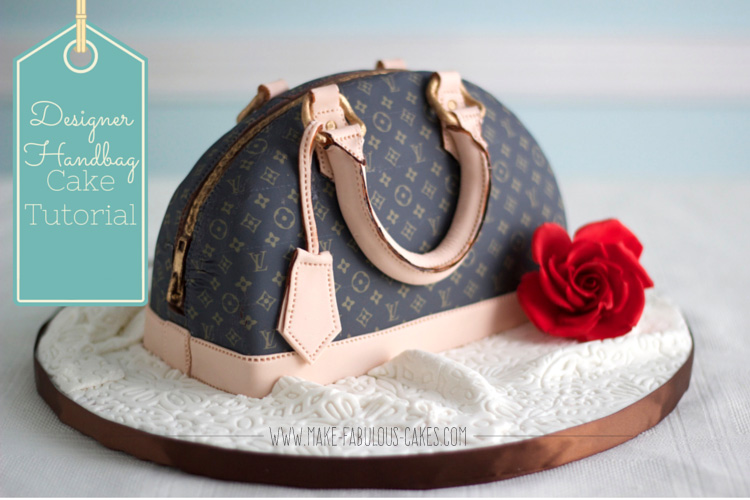In this image, we see a meticulously crafted cake designed to look like a Louis Vuitton handbag. The cake, resembling a small, hand clutch purse, sits atop a white lace doily on a circular brown platter. The handbag cake features the iconic Louis Vuitton logo, a gold arched zipper, and pink trim with peach-pink handles. A red rose is placed next to it, adding a touch of elegance. The setup rests on a table covered with a white tablecloth, with a light blue background that is slightly out of focus, keeping the attention on the cake. To the left side of the image, there is a teal green tag that reads "Designer Handbag Cake Tutorial," emphasizing the instructive nature of the image. Additionally, the website MakeFabulousCakes.com is subtly superimposed at the bottom, providing a source for further exploration. The detailed decor and realistic design make it initially appear as an actual handbag until closer inspection reveals it to be an expertly designed cake.